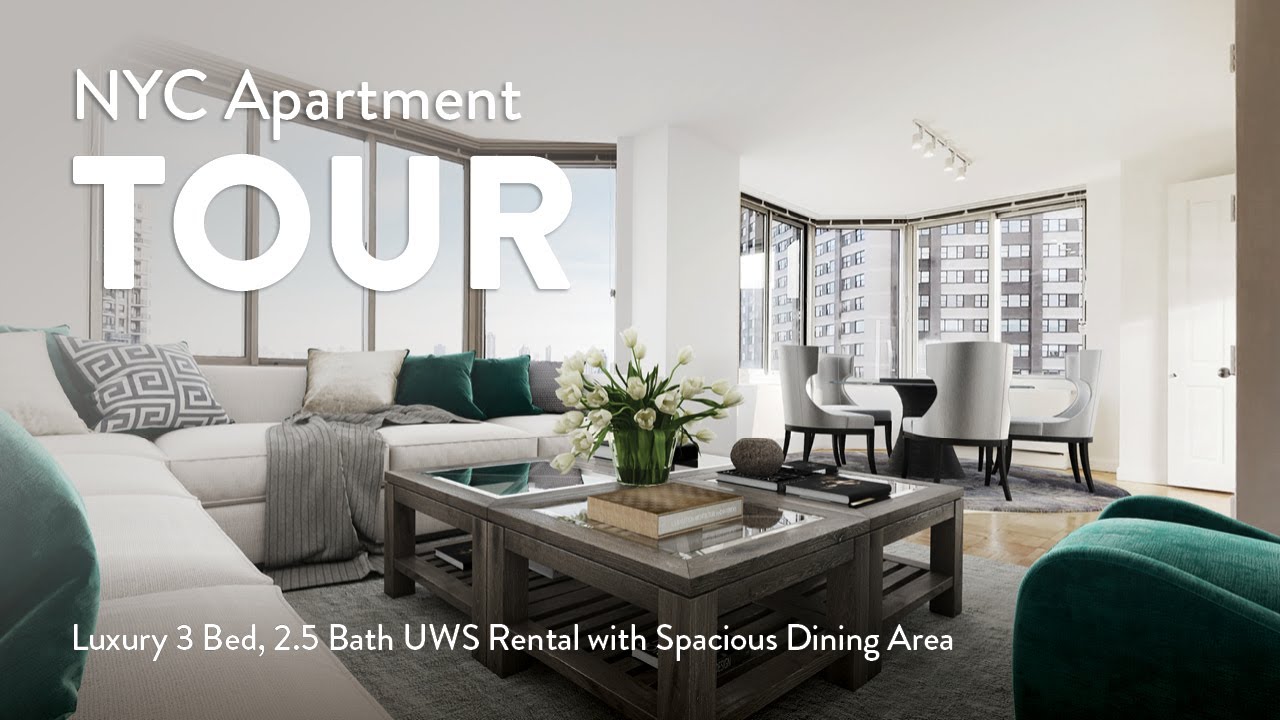This image showcases a luxurious New York City apartment, specifically labeled as a "New York City apartment tour." The apartment is bathed in natural light from large windows on the left side and extending towards the right, offering a panoramic view of the city's skyline. The interior predominantly features a white color palette, from the walls to the ceiling lights, creating a bright and airy atmosphere. 

A striking L-shaped couch defines the living room area, complemented by coffee tables adorned with books and a charming bouquet of white flowers. The comfortable setting also includes an elegant high-back, padded chairs gathered around a glass dining table situated near the expansive windows. This dining area not only promises a captivating view of the city's towering buildings but also rests upon an area rug that adds an element of coziness to the space. 

On the lower part of the image, a discreet white text announces the apartment as a "luxury 3 bed, 2.5 bath UWS rental with spacious dining area," highlighting the upscale nature of the property. Further down, the living room is accentuated by another area rug, tying together the aesthetic and functional elements of this sophisticated urban residence.